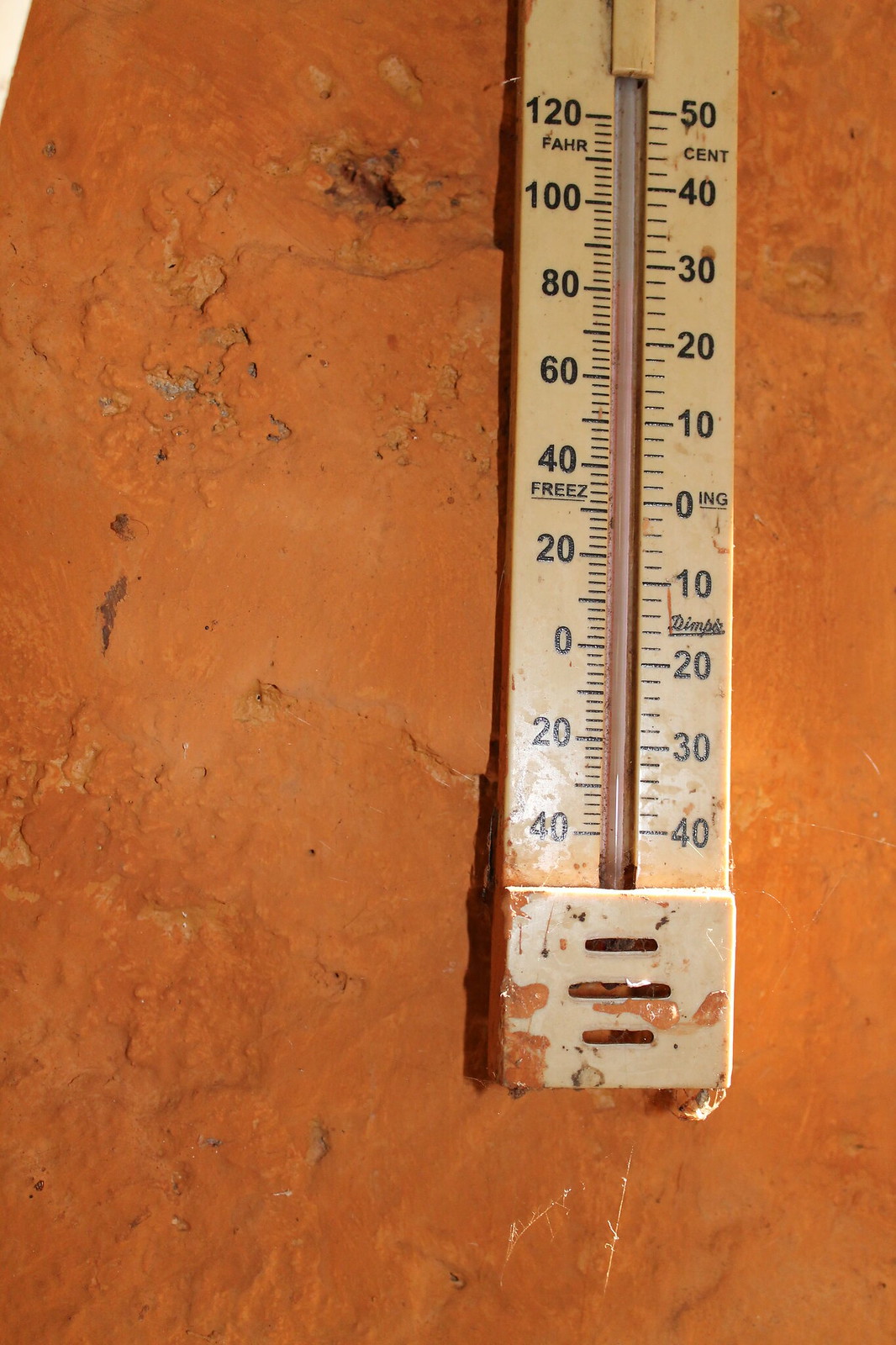The image is a first-person perspective shot capturing an old, discolored outdoor thermometer mounted on a rugged brown cement wall. The thermometer itself is yellowed with age and marred by numerous brown splotches on its cover and frame, giving it a weathered and neglected appearance. Its design is rectangular and elongated, reminiscent of a ruler. The white frame of the thermometer features a dual-scale display: Celsius readings on the right and Fahrenheit on the left. The Celsius scale ranges from -40 to 50 degrees, while the Fahrenheit scale extends from -40 to 120 degrees. Positive temperatures are displayed at the top, and negative temperatures at the bottom.

The wall to which the thermometer is attached appears to be painted concrete, although the paint is heavily worn and chipped. The surface is marked by scratches, notches, and various imperfections, suggesting a long tenure exposed to the elements and possibly inadequate maintenance or repair. The overall scene evokes a sense of rustic abandonment and tells a story of long-term exposure to weather and time.